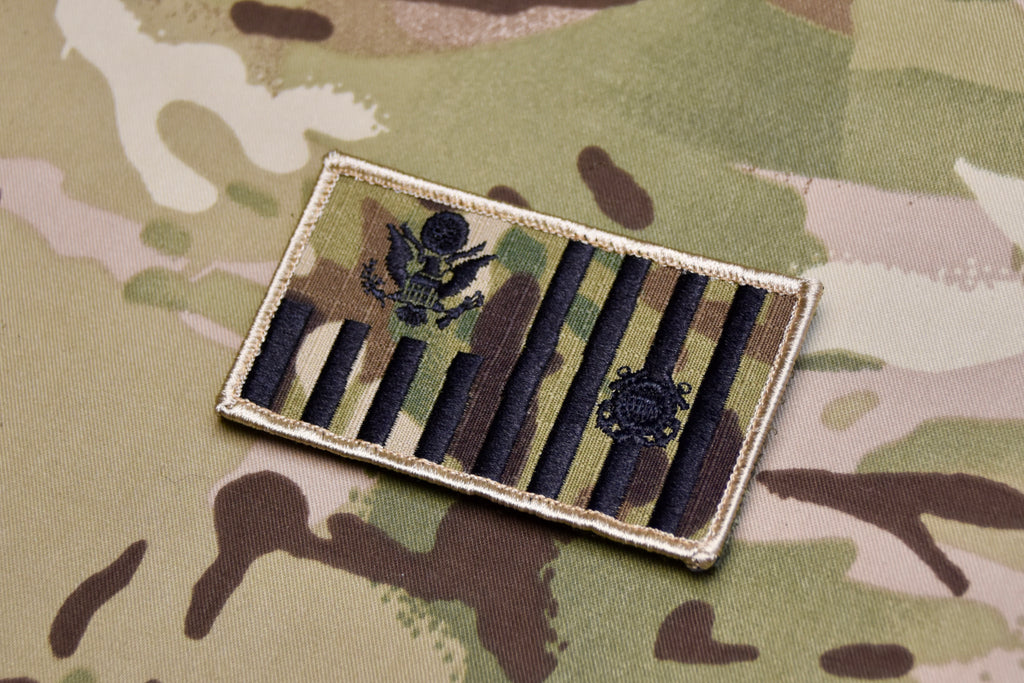This image is a close-up of a military patch affixed to a camouflage military uniform. The camouflage background features a typical pattern with colors including dark brown, white, tan, and various shades of green. The patch itself is rectangular in shape and prominently bordered with golden embroidered thread. The patch's intricate design includes numerous vertical black embroidered lines; most of these lines extend from the bottom of the patch, with some reaching the top and others stopping halfway up. The top left quadrant of the patch depicts a black eagle clutching a shield, branches, and arrows, indicative of a military emblem. The other quadrants primarily consist of vertical black bars, among which one section is adorned with a barely distinguishable seal, likely representing various branches of the military.